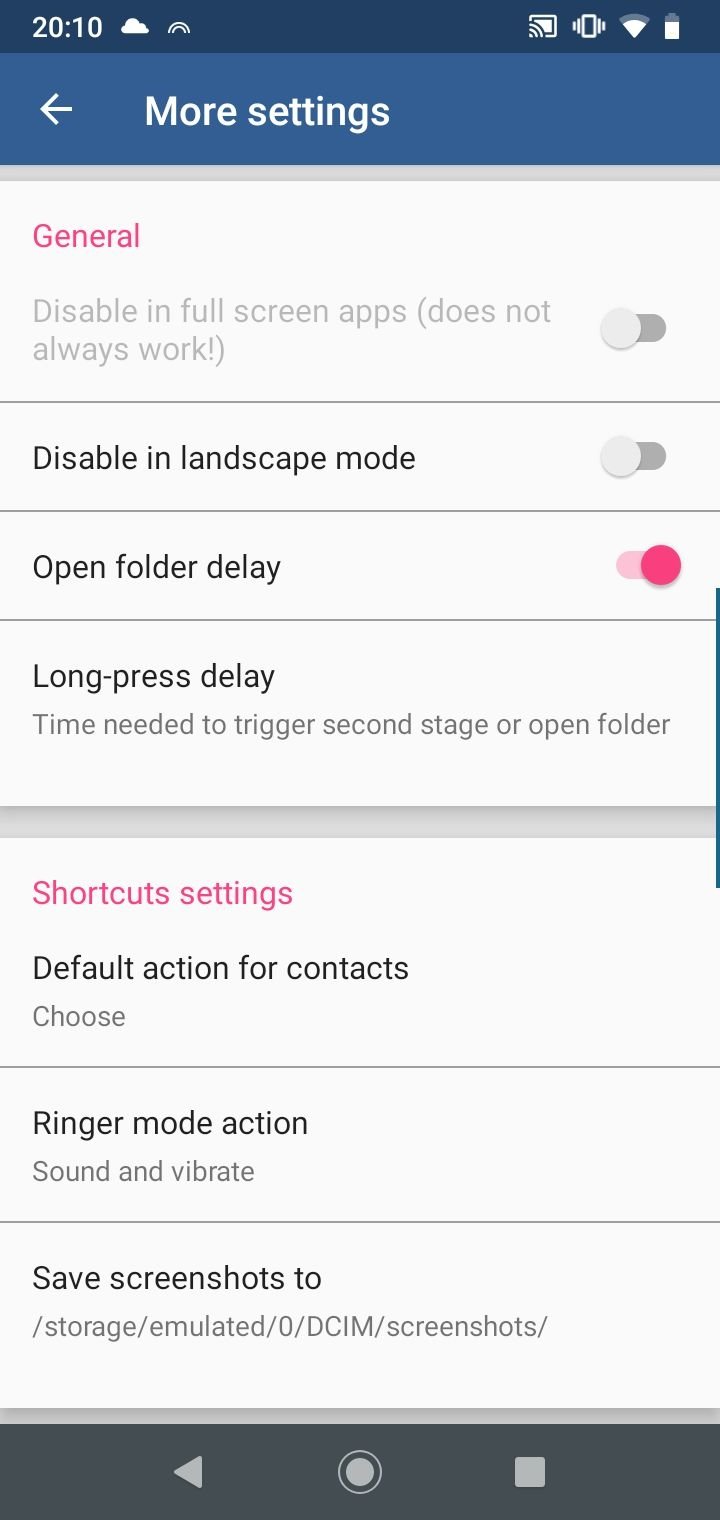A cell phone screenshot displaying a settings page:

At the top of the screenshot, there's a dark blue header with the text "2010". Below that, an image of a cloud and a rainbow is depicted. The status bar shows several icons: a screencast icon, a vibrate mode icon, mostly full cell reception bars, WiFi coverage bars, and a mostly full battery icon.

Beneath the header, there's a lighter blue bar with a white arrow pointing to the left, labeled "More settings". The main content section has a whitish-gray background with gray text.

The first section is titled "General". Underneath, a setting reads "Please disable fullscreen apps, does not always work" with a slider next to it positioned to the left, indicating that it is turned off.

Next, there is a black text label "Disable landscape", also with a slider to the left, indicating it is turned off. Following that is "Open tray folder delay", which has a pink slider positioned to the right, meaning it is turned on. Below this, it explains, "Long press delay: time needed to trigger second stage or open folder".

Further down, there’s a subtitle in black text, "Shortcuts and Settings". Under this, various settings include:
- "Default action for contacts: Choose"
- "Ringer mode: Sound and vibrate"
- "Save screenshots to: /storage/emulated/0/DCIM/screen//"

At the bottom of the screenshot, there is a darker gray navigation bar with three icons: an arrow pointing to the left on the left side, a circle in the center, and a square on the right side. These icons are in a lighter gray color.

Note: The last part of the original caption contained inappropriate language and irrelevant remarks, which have been omitted for clarity and appropriateness.